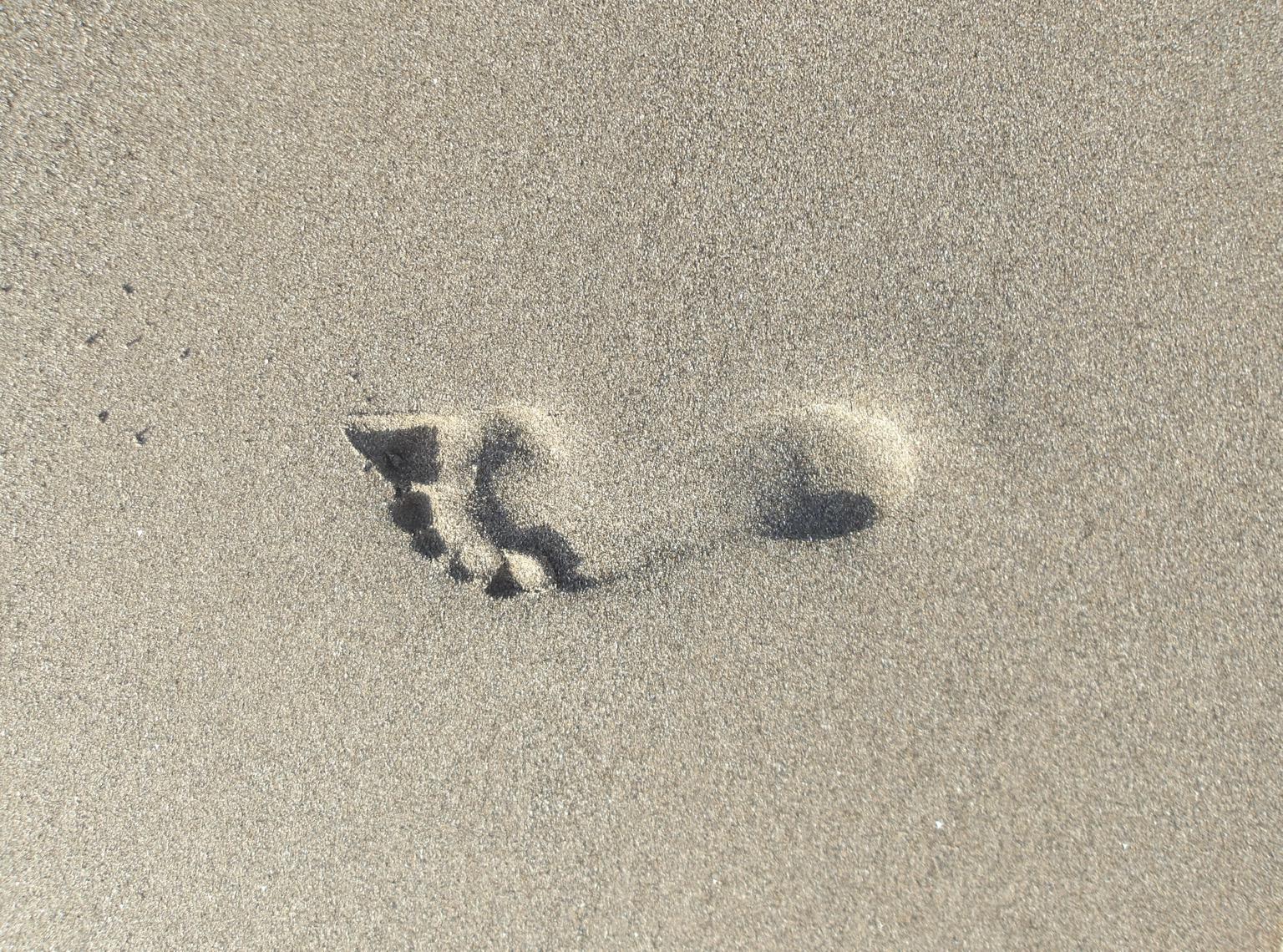A meticulously captured color photograph showcases a single, pristine footprint embedded in fine grain sand. Positioned in the direct center of the image, the footprint faces with the toes pointing towards the left center. It's a left foot, characterized by a strong curve and slender form, suggesting a larger yet narrow size. Sunlight illuminates the sand, creating intricate shadows around the outer heel, the top region near the toes, and the curve beneath the toes. The arch on the left side blends smoothly with the surrounding sand, creating a seamless and natural impression. Light highlights accentuate the contours, particularly on the outer heel and along the top where the big toe lies, adding depth and dimension to the serene scene.